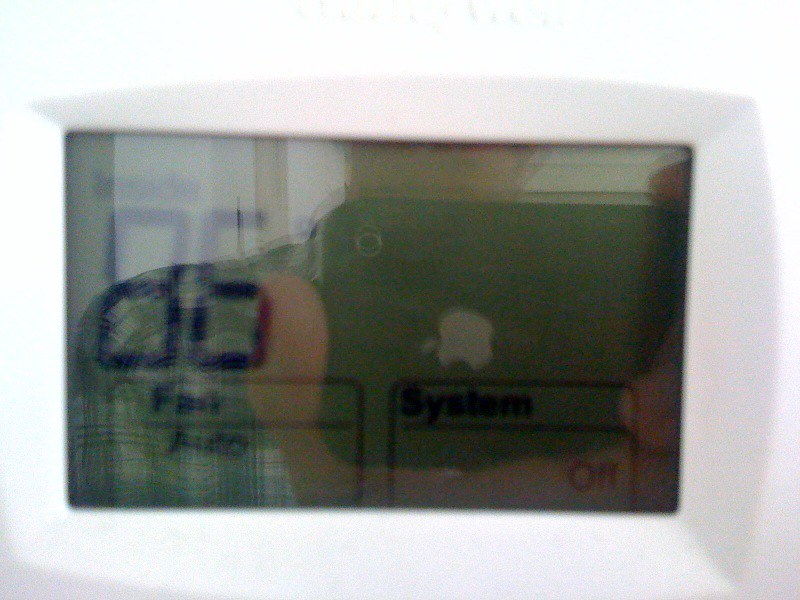The image is a stark white expanse, presenting an intriguing ambiguity where neither objects nor background distinguish themselves. It evokes a minimalist aesthetic, inviting viewers to interpret its blankness. Whether an error or an intentional canvas for mental projection, this image leaves ample room for personal reflection. Imagining my own life's overwhelming demands—ranging from professional responsibilities to intricate personal tasks, my son's educational and extracurricular activities, and summer planning—this blankness transforms into a chaotic, vibrant swirl of colors and forms, symbolizing the teeming chaos that often populates my mind.